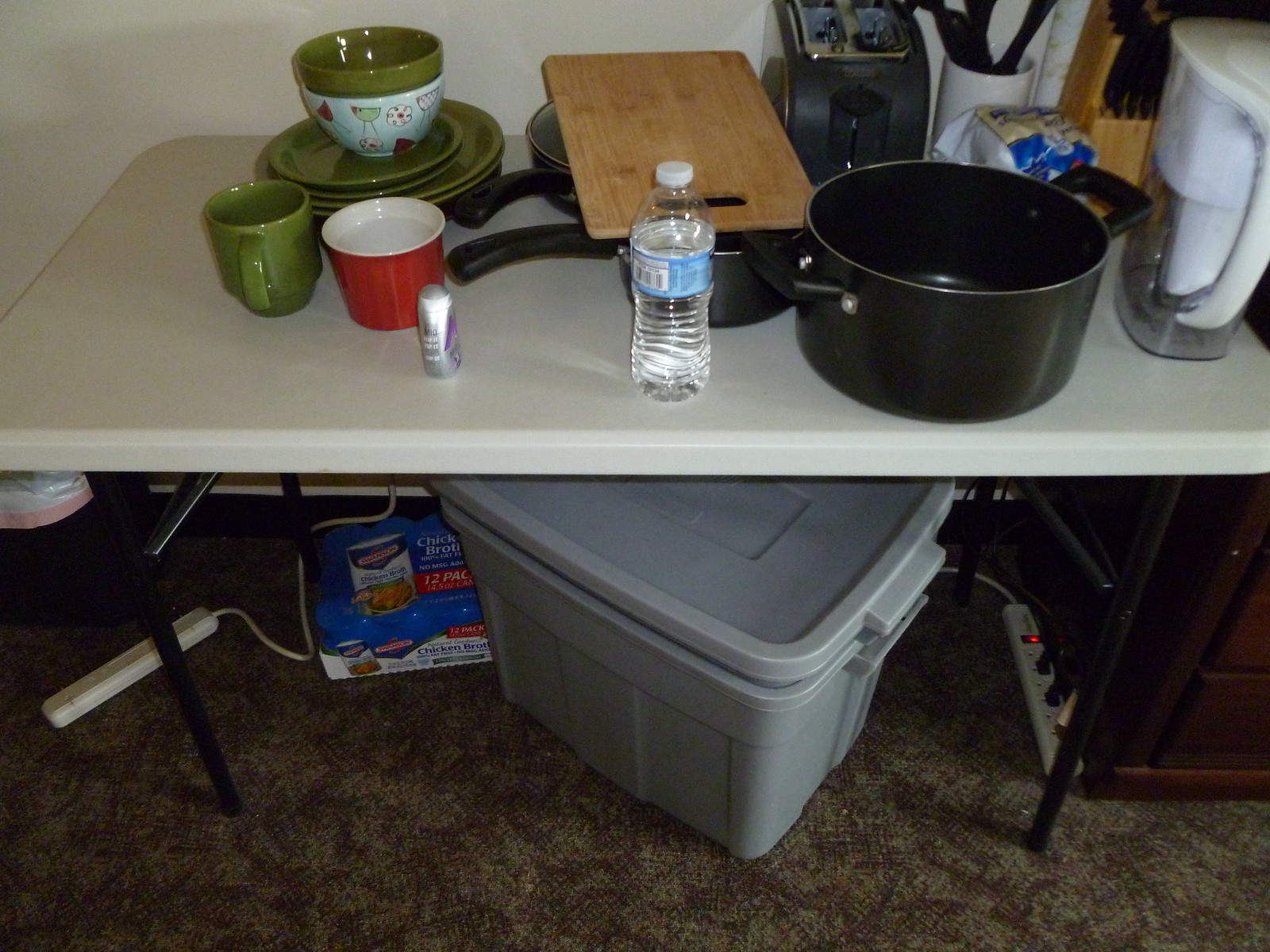This indoor color photograph captures an overhead view of a white folding table positioned against a white wall. On the tabletop, from left to right, several green, round dishes are neatly stacked with a white-patterned saucer on top of the pile. In the foreground, there are two cups: a green cup on the left and a red cup on the right. 

To the right of the cups, two pots are placed side by side with their handles jutting out to the left, partially covered by a rectangular cutting board whose handle points towards the photographer. In front of the cutting board, a full 12-ounce white plastic water bottle with a clear cap and a blue label rests on the table. 

Further to the right, a large, seemingly new cooking pot sits behind the water bottle. Next to this pot, and against the wall, is a two-slice toaster. Directly to the right of the toaster, a ceramic cup holding a cluster of black utensils is placed, although the tops of the utensils are cut off by the frame. To the far right of the table, there's a water pitcher with its handle facing the camera, and behind it, a wooden knife block is visible.

Beneath the table, behind its left leg, there's a rectangular outlet with a cord that trails off to the right and disappears under the table. To the right of the outlet sits a box, presumably food packaging, adjacent to a large gray plastic tote with a slightly askew gray lid, seen from a three-quarter perspective. Further to the right, a power strip with an illuminated indicator light is visible, accommodating three or four plugged-in devices. 

The foreground features a dark brown carpet, and no text or print is legible in the photograph.